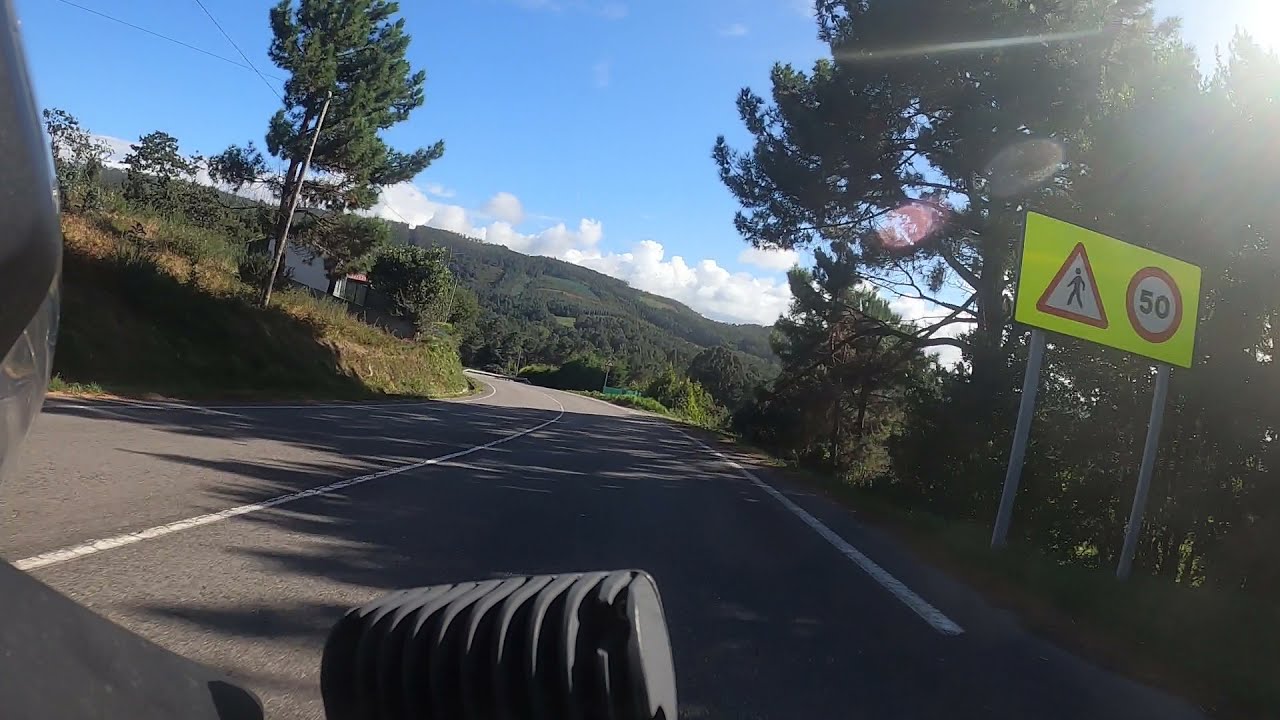This image captures the first-person perspective of someone riding a motorcycle down a winding rural road on a sunny day. The road, painted grey with white lane markings, curves gently to the left and continues into a lush landscape dominated by hills. On the right side, a bright yellow sign held up by two steel beams displays a red and white yield symbol and a speed limit of 50 within a red circle. The right side of the road features a mix of multiple tall trees and grass-covered ground, along with a sharp drop-off descending down a hill adorned with green shrubbery. The left side similarly displays a field dense with tall trees, grass, and some dead weeds, leading upward into more hills covered in vibrant greenery. The scene is bathed in sunlight, with shadows cast onto the road by the surrounding trees. High above, the sky is a rich blue, accentuated by a few scattered white clouds near the horizon, indicating the image was taken during the day. In the foreground, part of the motorcycle—possibly the helmet and headlamp—is visible, confirming the mode of travel.